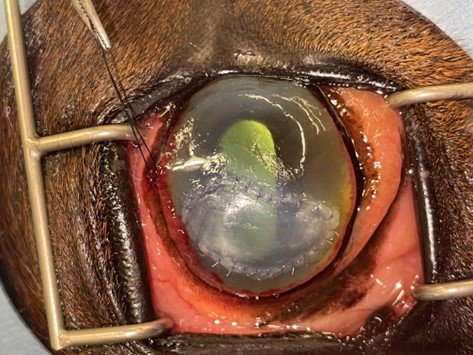This detailed close-up depicts a surgical procedure being performed on what appears to be an animal's eye, possibly a horse. The eye, which has a green center, is held open by two brown metal brackets, revealing the pink flesh of the surrounding eyelid. The area around the eye is framed by brown fur with slight hairs. 

In the upper left of the image, a pair of needle-nose pliers holds a piece of black thread, which is being used to apply stitches around the inside of the eye. The eye itself shows red veins and a mix of red and black areas, suggesting previous incisions or repairs. The use of various tools and the presence of multiple stitches indicate an ongoing or complex operation, possibly similar to LASIK surgery.